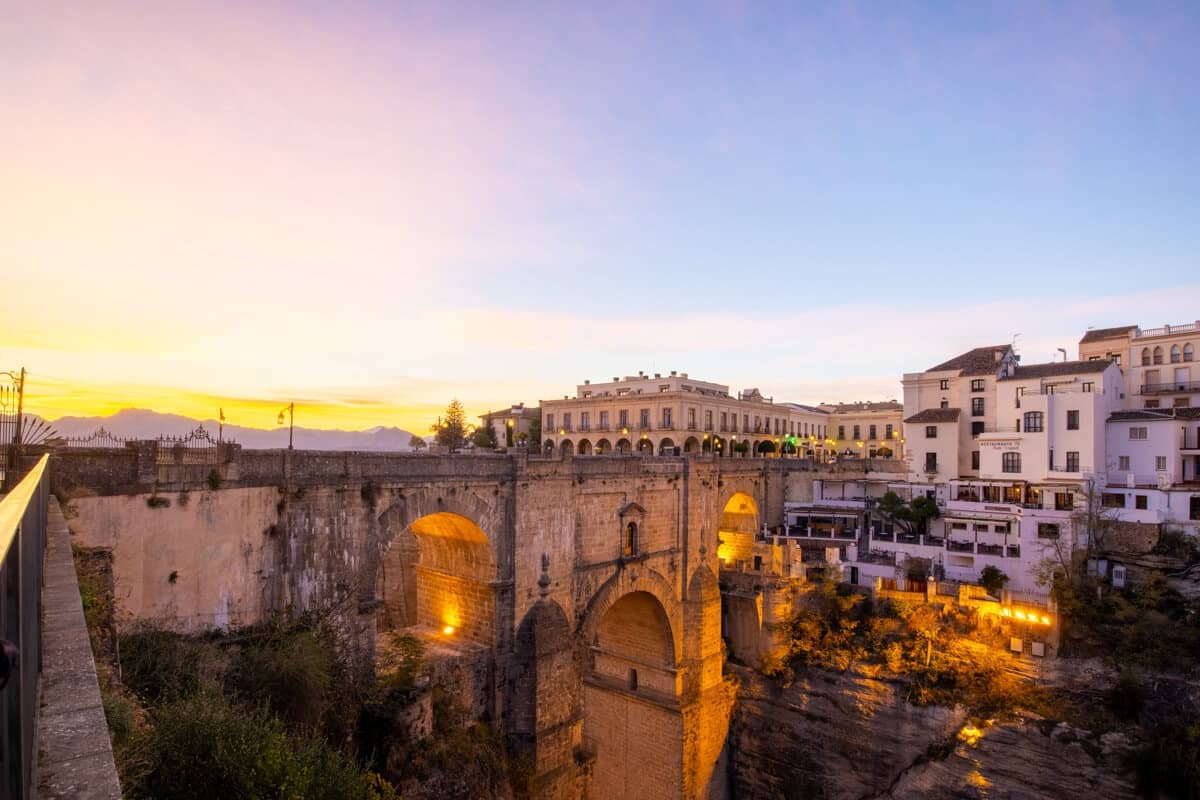This photograph captures the picturesque scene of a European city at sunset. In the foreground, an old stone bridge, built into a cliff, stretches from the left to the right side of the image. The bridge, crafted from tan stone, is illuminated by warm yellow lights underneath, enhancing its historic allure. Below the bridge, the cliff's edge limits the view to the bottom.

In the background, white buildings cascade down the cliffside, each story sloping toward the edge. These tall structures are complemented by additional tan stone buildings, all adorned with yellow lights that create a welcoming glow. To the left, the setting sun casts a golden hue over the lower part of the sky, transitioning to a serene blue on the right, punctuated by scattered clouds. Distant mountains form a majestic backdrop, completing the timeless charm of this European urban landscape.